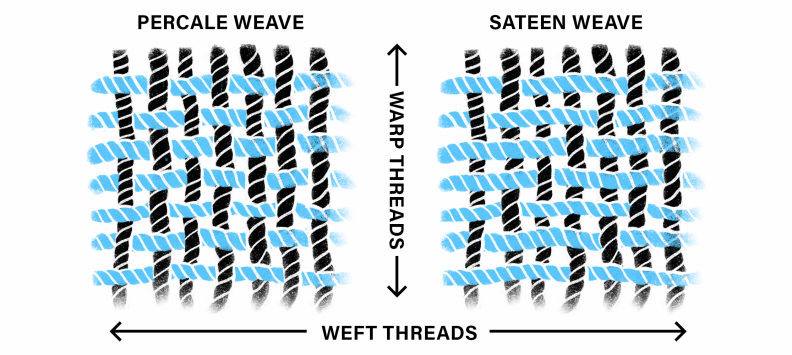This image illustrates two different types of weaves: percale on the left and sateen on the right. Both sections feature interwoven threads with black warp threads running vertically and light blue weft threads running horizontally. The text "percale weave" is positioned at the top left above a standard weaving pattern with an alternating over-under structure. On the right, "sateen weave" is labeled above a more irregular pattern where weft threads pass over multiple warp threads before going under one. Separating the two illustrations is the text "warp threads," written vertically with corresponding arrows pointing up and down, while at the bottom middle, the label "weft threads" includes arrows pointing left and right, emphasizing the threads' directionality in the weave patterns. The background of the image is white, making the black and blue threads, as well as the white spirals denoting their texture, distinctly visible.